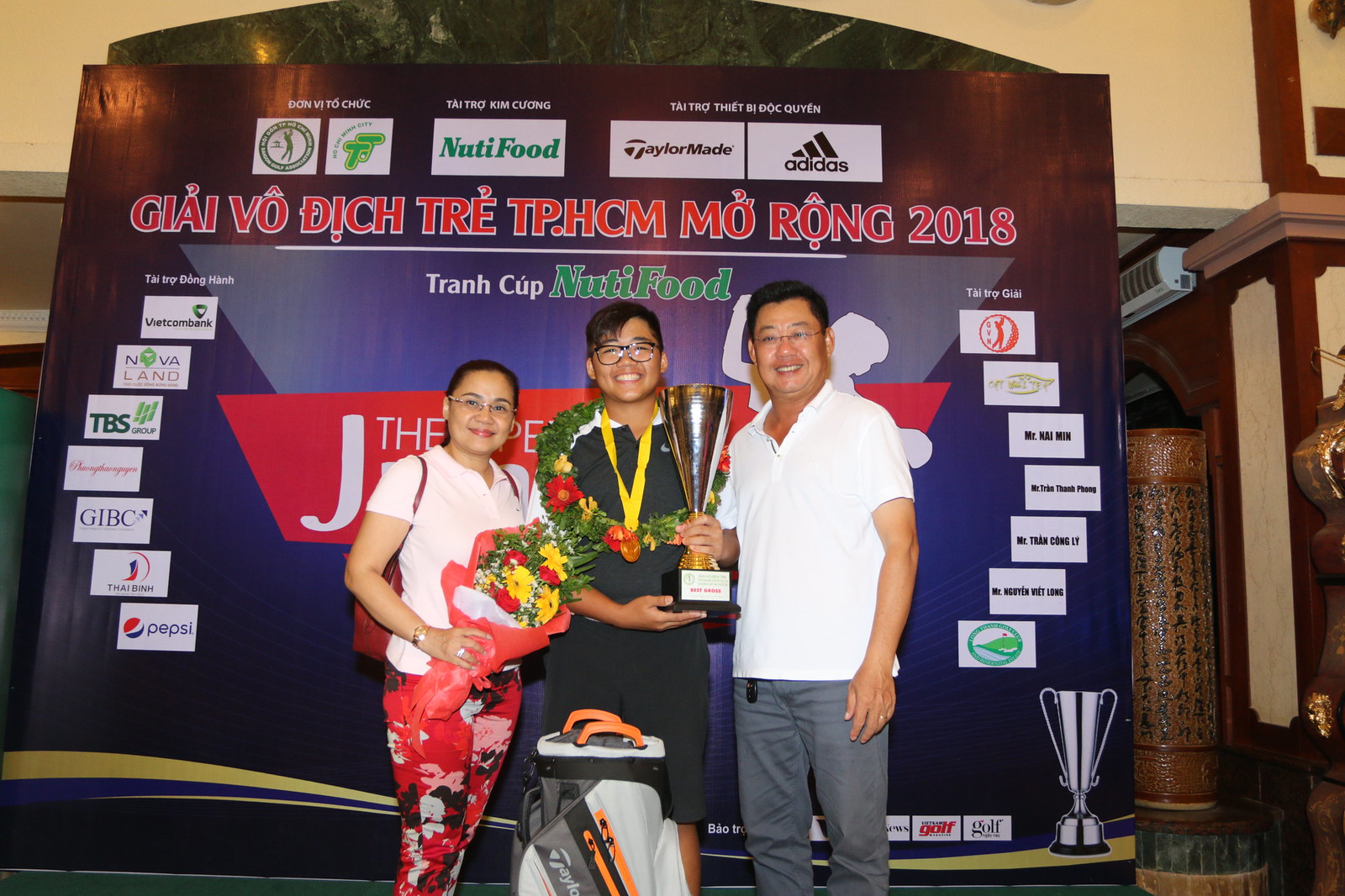This press photograph, likely from a golf event in Asia—perhaps the Philippines or Vietnam—features a young man in his late teens or early 20s standing proudly in front of a ceiling-to-floor banner adorned with logos of sponsors like Pepsi, TaylorMade, Adidas, and Nutty Food, indicating it is the Trang Cup of 2018. The young man, who is wearing a black-and-white polo shirt, black pants, and black-framed glasses, smiles broadly as he holds up a cone-shaped golden trophy with a black base. Draped in a green floral lei and adorned with a bronze medal on a yellow lanyard, he stands between his parents. To his left, his mother, with black hair pulled back and wearing glasses, sports a white polo shirt and vibrant floral print pants, while holding a bouquet of red and yellow flowers wrapped in red paper. To his right, his father, also bespectacled with dark hair, is in a white polo shirt and grey pants, smiling proudly. At the bottom, a TaylorMade golf bag is partially visible, corresponding with the golf theme suggested by the trophy and attire. The backdrop, with red and green text, is set in what seems to be a convention room or possibly a temple, adding to the celebratory yet formal ambience of the event.